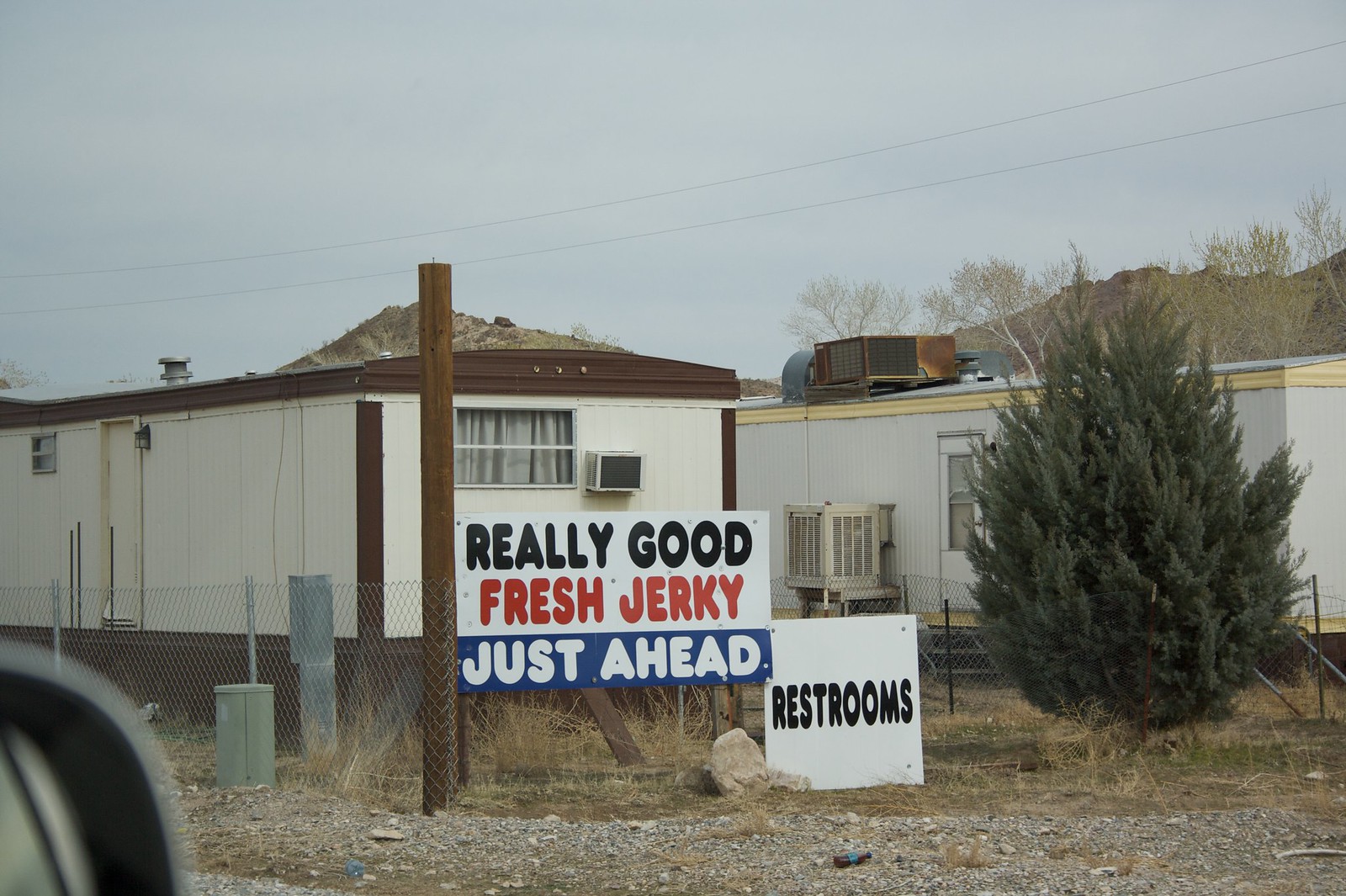This landscape photograph captures a rustic roadside scene. Dominating the center is a prominent sign that reads "Really Good Fresh Jerky Just Ahead," while slightly lower and to the right, another sign indicates the location of "Restrooms." The setting includes a few mobile home trailers surrounded by simple fencing, with air conditioners visible on the structures. In the background, rolling hills or small mountains stretch across the horizon under a clear sky. A tall pine tree stands prominently on the right-hand side of the image. The photograph appears to have been taken from inside a vehicle, as the shape of a car mirror is visible in the lower left-hand corner. The colors in the image include various shades of brown, white, cream, green, black, red, and blue.